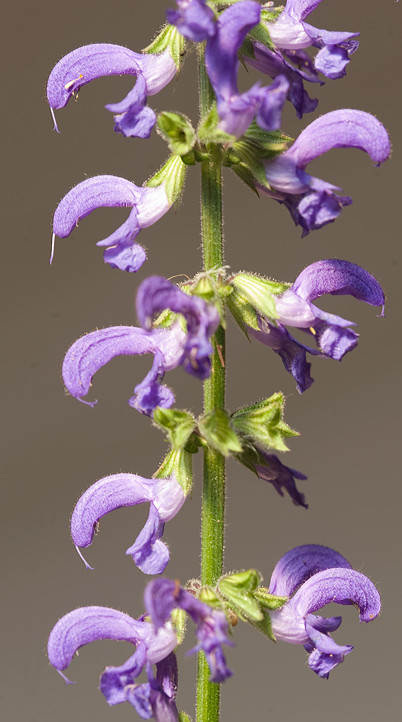The image features a vibrant, light purple flower with multiple blossoms growing from a green stalk. Each blossom emerges from a green base, and the flower's arrangement is almost symmetrical, with five blossoms on the left side and four on the right, suggesting one may have fallen or been plucked. The blossoms have a unique shape with a prominent central arm and a smaller beak-like structure extending over the top. The stem shows a texture of fine fuzz typical to some flower stalks. The photograph has a minimalistic backdrop, in shades of gray, which highlights the delicate beauty and detailed structure of the flower. The setting emphasizes the flower's graceful form and the soft yet striking color palette.